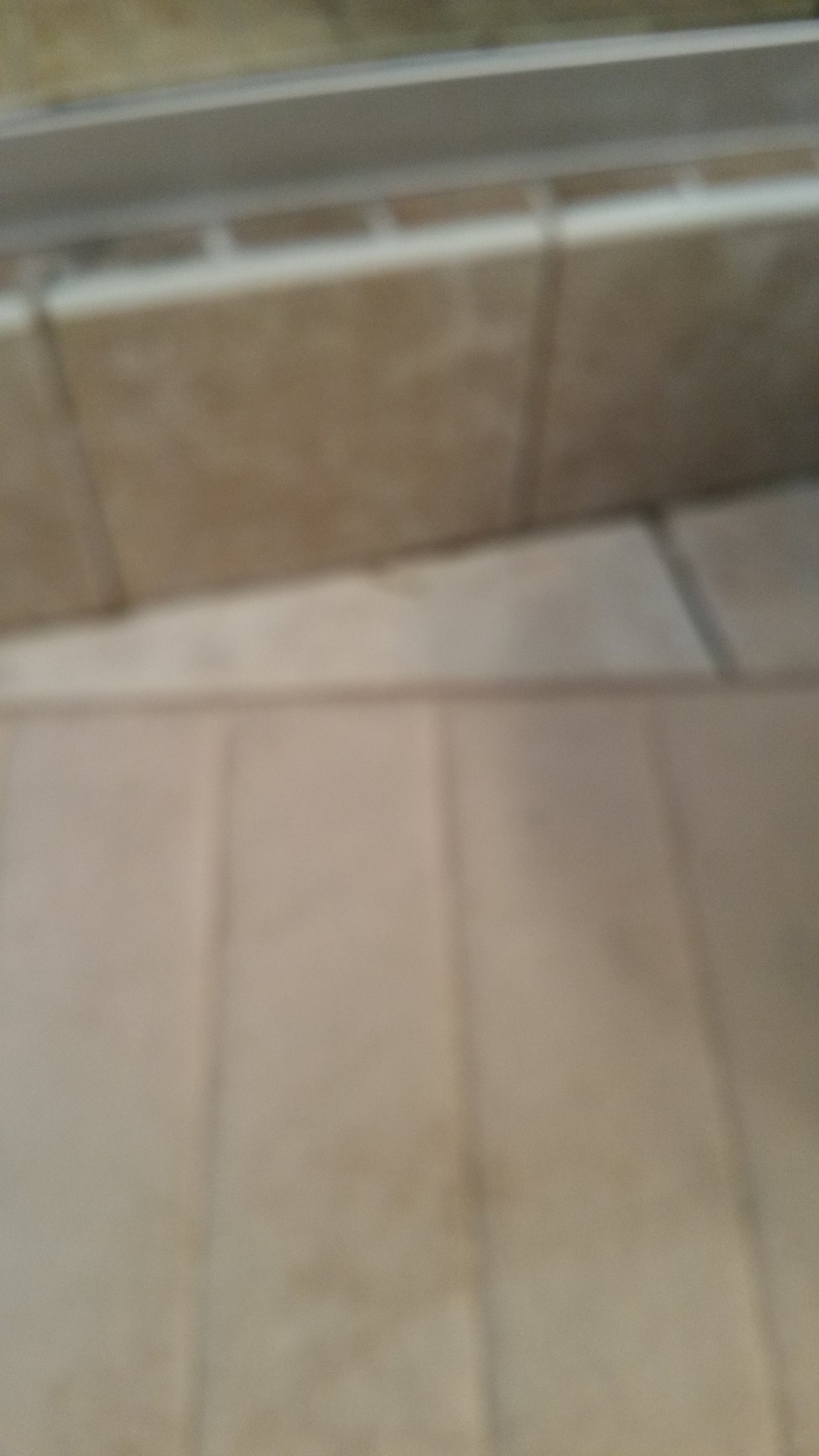This color photograph, though slightly blurry and out of focus, vividly captures the bottom two-thirds of what seems to be a concrete or possibly stone walkway. The surface is a grayish hue, and clear demarcations between the slabs of concrete or stone are visible, adding texture and dimension to the scene. In the upper section of the image, a stone railing is discernible despite the blur. The beautiful stonework exhibits light brown tones interlaced with touches of gray, hinting at its intricate craftsmanship. Atop the stone railing sits a metal component, likely made of steel, showcasing a dull silver finish. Together, these elements create a fascinating interplay of materials and colors, despite the photograph's lack of sharp focus.